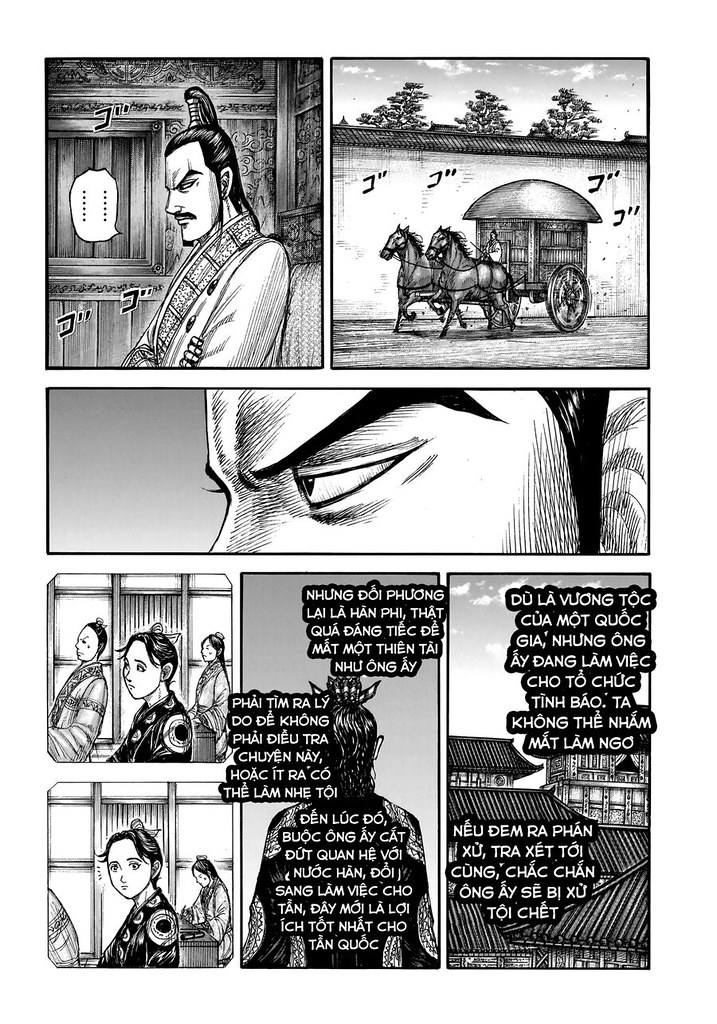In this black, white, and grayscale comic strip, we follow the narrative through several well-detailed panels. The first panel introduces a stern-looking man with traditional Japanese Samurai attributes – slicked-back hair tied up in a ponytail, dramatic eyebrows, and facial hair – seated in a room. Beside him, we see a carriage drawn by two horses set against a backdrop of trees. This scene transitions to an eye-catching close-up of the man’s intense, contemplative gaze. Further down, a young girl appears in two expressive panels, displaying concern and deep thought, with other women slightly visible in the background. Finally, the scene shifts to the back view of the primary Samurai character standing outside a house. The context remains elusive as all text is written in a foreign language, heightening the enigmatic and solemn ambiance of the comic.